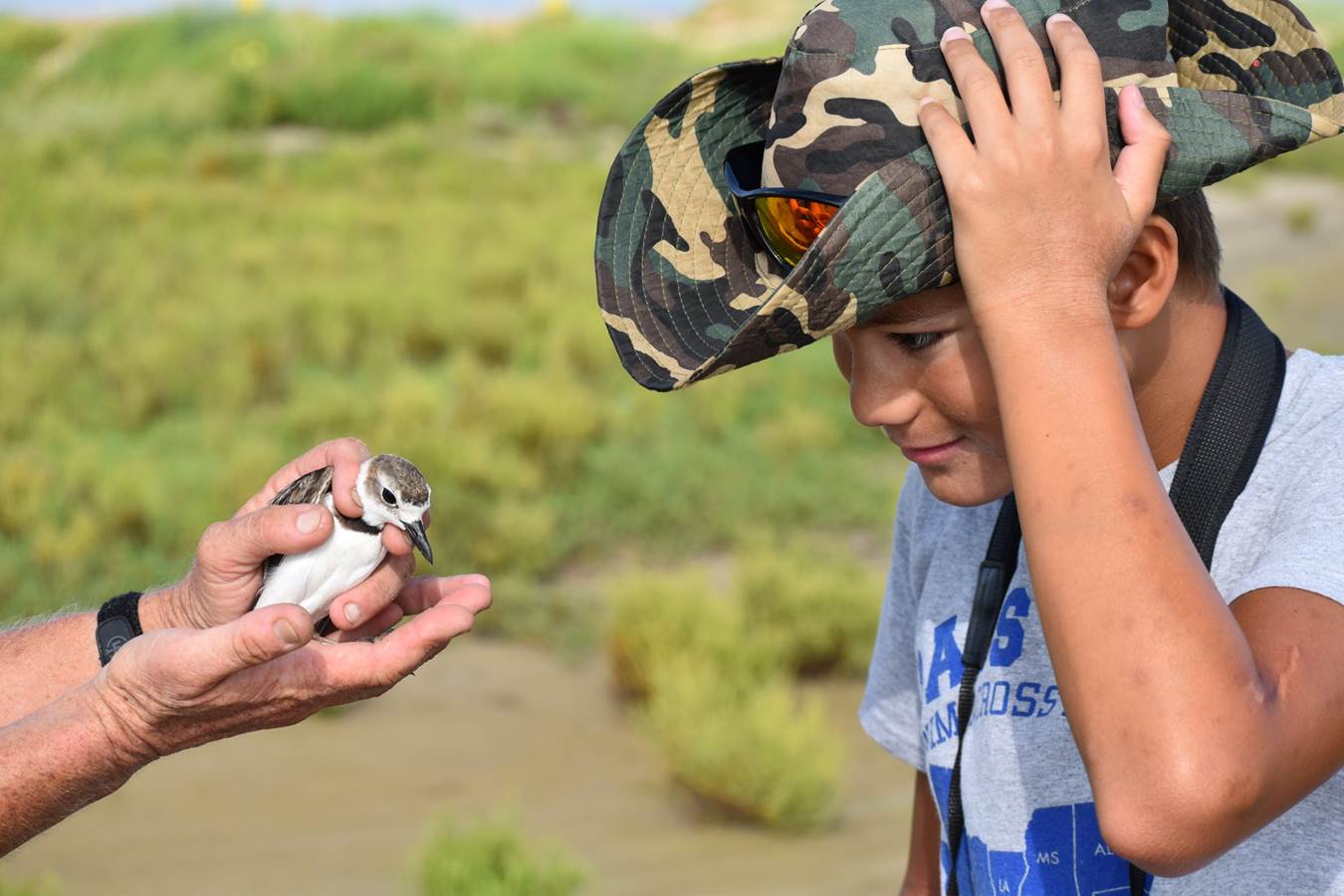This photograph captures a young boy, likely around 10 years old, enjoying a sunny day outside. He stands on the right side of the image, looking towards the left at a bird that someone is holding. The boy, who has slightly tan skin, wears a white t-shirt and a camouflage jungle-style hat adorned with sunglasses on the front. His left hand is touching the brim of his hat, and he is smiling. The bird in the photo has a predominantly white body with light brown on its head and a small black beak. The person cradling the bird has visibly wrinkled arms, adorned with a black watch band, suggesting they might be elderly. The background showcases a vibrant green lawn with a few light green bushes scattered throughout the scene. The photograph is horizontal and rectangular, capturing this serene moment in great detail.